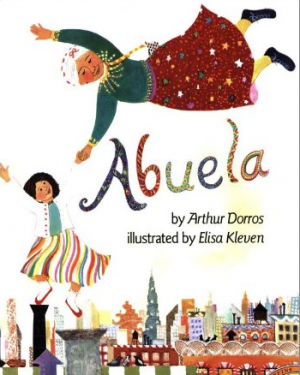The image is a vibrant children's book cover titled "Abuela," with colorful letters spelling out the title across the middle. Below the title, in black text, it reads, "by Arthur Doros, illustrated by Elisa Clevin." The cover is set against the backdrop of a bustling city street with a variety of buildings lining the bottom. On the left-hand side, a little girl with black hair is standing on a rooftop. She is dressed in a white top, a colorful skirt, white socks, and orange ballet slippers. Her arm stretches upward towards an older woman. The older woman, or "Abuela," appears at the top right of the cover, seemingly flying. She is adorned in a red star-patterned skirt, a green sweater, yellow stockings, black boots, and a colorful turban. Both characters are animated and joyful, capturing a sense of adventure and whimsy.